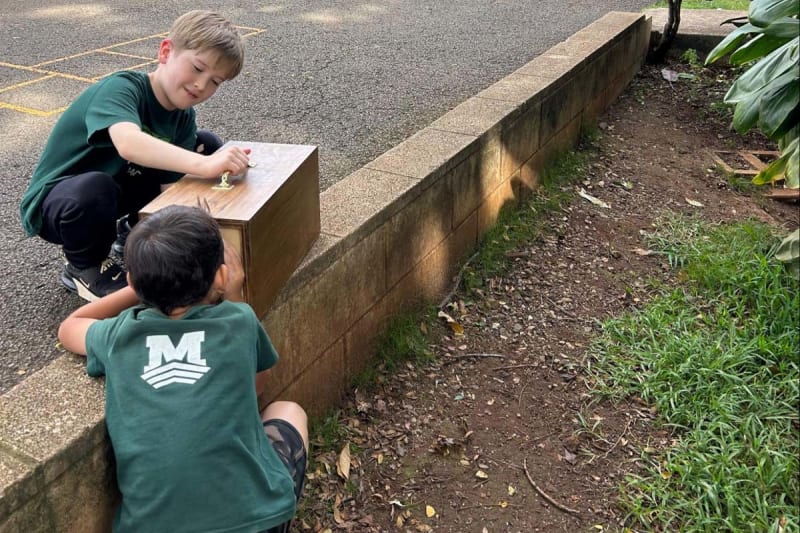In this detailed photograph, we see two boys engrossed in play around a wooden box with a golden handle, positioned atop a small two-foot brick stoop. The boy on the left side of the picture, who appears to be around 11 years old, has sandy blonde hair and is dressed in a green t-shirt and black jeans, along with black shoes. He is grasping the handle of the wooden box with his right hand. Meanwhile, the other boy, who has dark black hair, is positioned on the ground to the right of the box, looking inside it and pressing his face and hands against the box as if peering into it. He is wearing a green short-sleeved shirt with a white ‘M’ on the back and dark shorts. The setting is outdoors near a playground; the ground transitions from asphalt with a yellow hopscotch etching behind the blonde boy, to an area of brown dirt and sporadic grass tufts beside the dark-haired boy. A small portion of a tree is visible in the top right corner of the image, adding to the photorealistic quality of the scene.